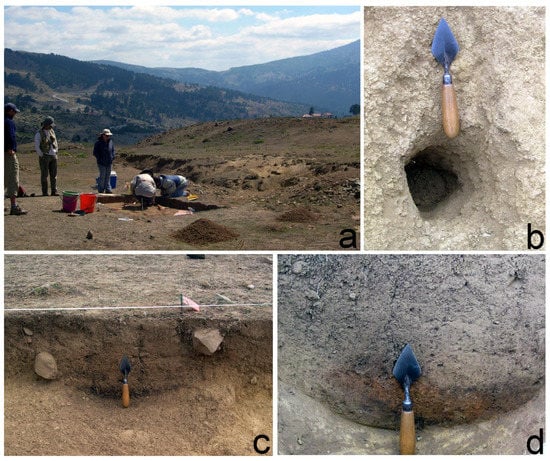This rectangular image is divided into four photographs labeled A, B, C, and D. Photograph A, the largest and positioned in the upper left corner, depicts a dry, hilly, and sparsely vegetated area under a blue sky with white clouds. Several people are engaged in what appears to be either a campground activity or an archaeological dig, as they kneel over a shallow, rectangular excavation. To the left, a few buckets are visible, with three observers standing nearby, two facing away and one facing to the left.

Photograph B, located to the right of A and much smaller with a vertical orientation, shows a top-down view of a significant hole in a rock formation. A digging tool placed above the hole provides a sense of scale.

Photograph C, found at the lower left, offers another perspective of an opening in the ground. Here, a similar digging tool is used to illustrate the slit’s width and the land’s thickness, suggesting comparisons in the depth of excavation.

Photograph D, in the lower right, presents a simple image of a rocky area with a digging pick lying on the dirt, emphasizing the tools used in the excavation activities across the other photographs.